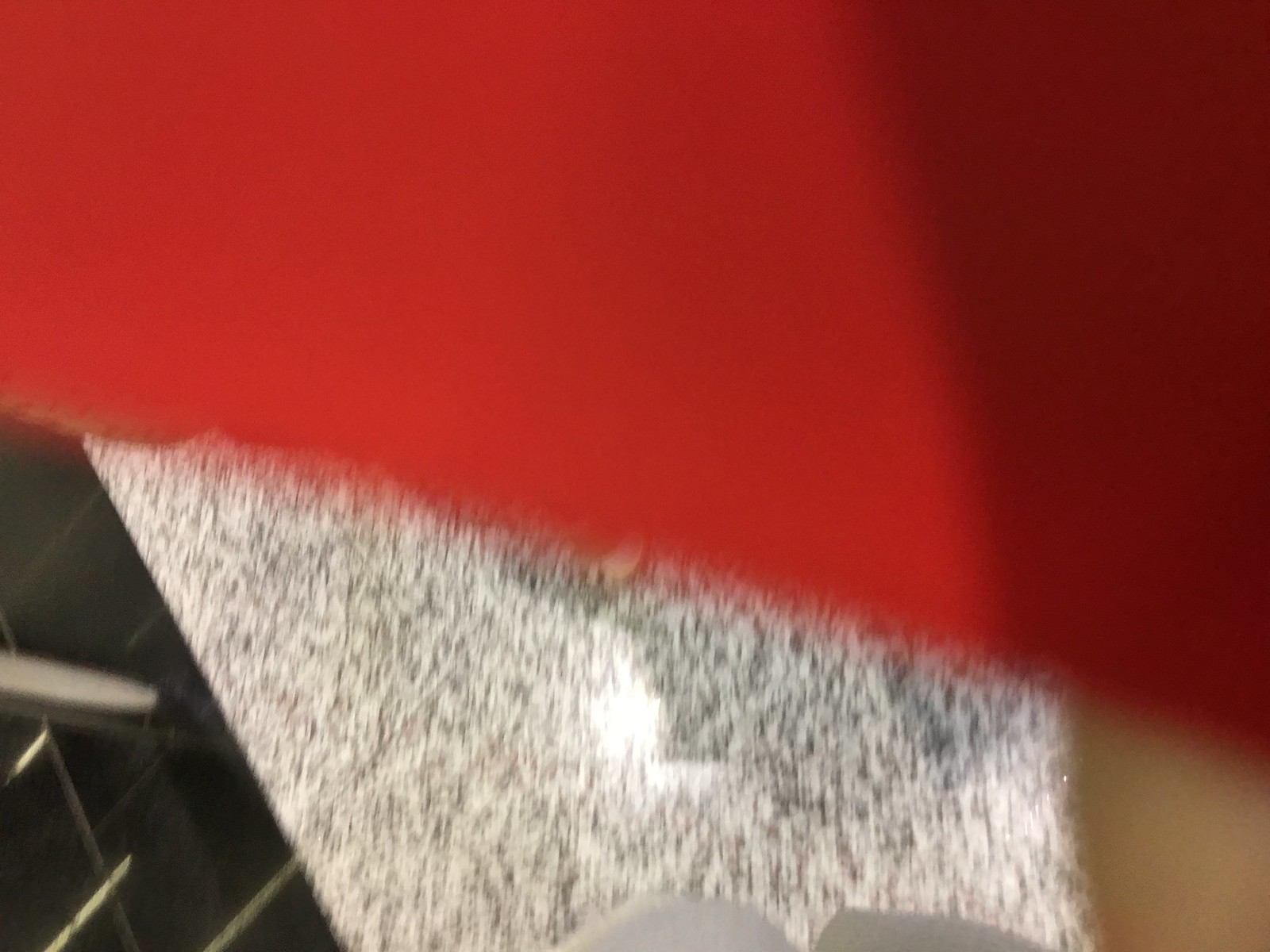This photograph captures a diverse array of objects and textures arranged in a seemingly casual yet intriguing composition. At the top of the image, a red object with a jagged lower edge, resembling a torn piece of paper, stands out prominently. Beneath this, a sliver of a yellow object peeks through, adding a contrasting pop of color. The floor features a patterned rug in shades of white, gray, and black, partly obscured but still noticeable. Just above this rug, there appears to be a person's knees, clad in white fabric, hinting at their presence in the scene. The floor below showcases sleek black tiles with light-colored grout, adding to the intricate details present in the photograph. A tall, skinny, silver object rests on the floor, catching the viewer's eye. The entire image is slightly grainy and features a light glare, giving it a textured and somewhat nostalgic look. Shadows cast on the red paper add depth to the composition, making the overall scene rich with visual interest and subtle interactions between the varying elements.